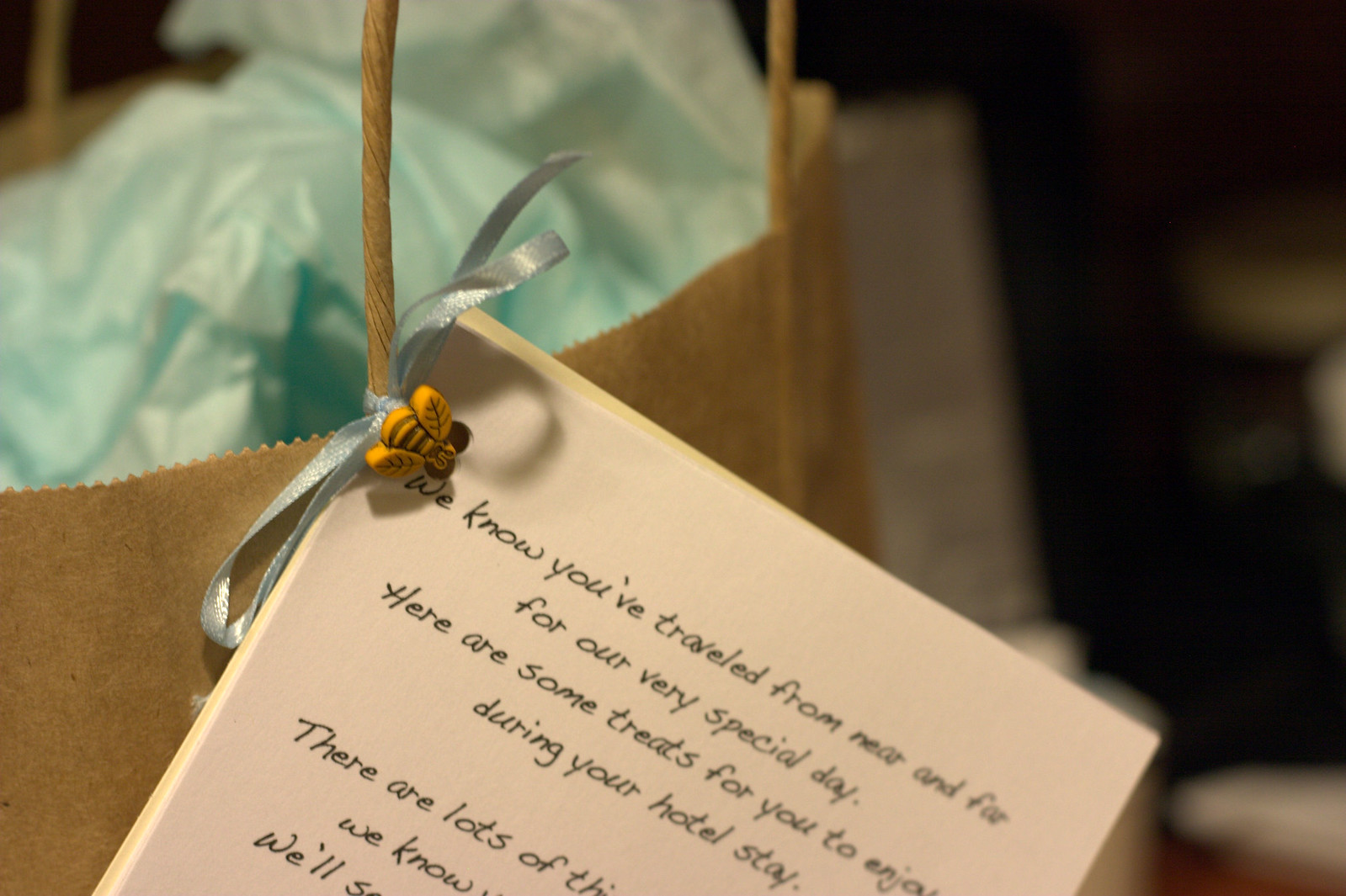This photograph depicts a welcoming gift bag situated in a hotel room. The brown paper bag contains blue tissue paper, suggesting the presence of gifts inside. The focal point is an elegant, white note with black text, which is attached to the bag's handle via a green ribbon tied to a small plastic yellow and black bumblebee. The note reads, “We know you've traveled from near and far for our very special day. Here are some treats for you to enjoy during your hotel stay.” The background appears to be the interior of a hotel room, although it is too blurry to discern specific details. This carefully arranged gift bag serves as a warm welcome to travelers, adding a thoughtful touch to their stay.